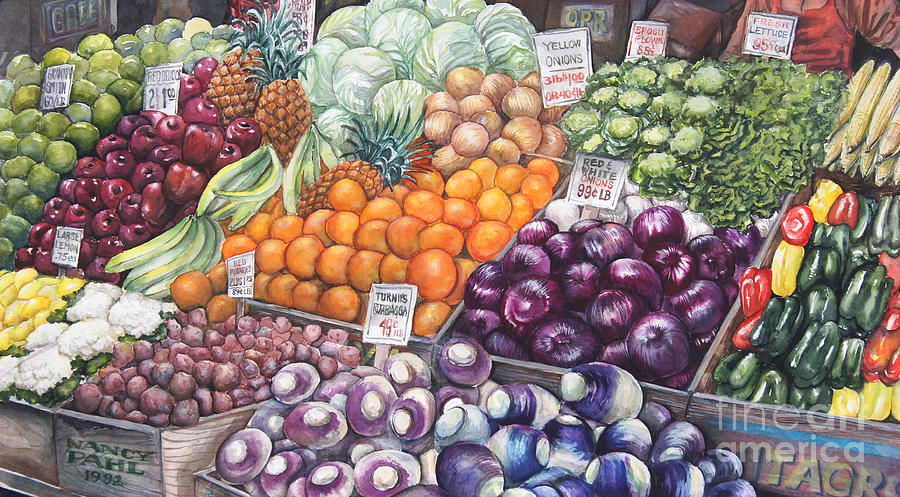This detailed painting captures the vibrant and bustling atmosphere of an outdoor farmer's market stand, showcasing an extensive assortment of colorful fruits and vegetables, each meticulously labeled with white signs indicating their prices. Central to the scene are crates and boxes filled with an abundance of fresh produce, including green apples, red apples, bananas, pineapples, lemons, cauliflower, red potatoes, oranges, kohlrabis, cabbages, Brussels sprouts, lettuce, corn, green, red, and yellow peppers, turnips, and various types of onions—white, red, and yellow. Some boxes are adorned with writing, while others are partially obscured by adjacent produce. Notable details include yellow onions priced at three pounds for a dollar and red and white onions at 99 cents per pound. Above the pepper crates lies corn with its yellow stalks, alongside artichokes. The vibrant composition is enriched with a variety of items, from mushrooms to exotic fruits. Signatures at the bottom indicate the artist as Nancy Fall, with the year 1992, and a Fine Arts America watermark marking the piece's authenticity.